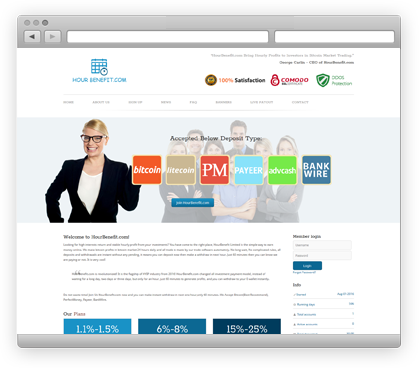The image appears to be a complex web page layout displaying various UI elements and icons:

At the top of the page, there is a gray border approximately an inch thick. In the top left-hand corner of this border, there is a gray circle, followed by another gray circle to its right, and then a slightly darker gray circle further to the right. Beneath these circles, there is a gray box featuring a black arrow pointing to the right. Next to this is another gray box with a slightly lighter gray arrow pointing to the right.

To the right of these gray boxes, there are two white boxes resembling search or address fields. Underneath these boxes, there is an image of a blue calendar icon with the text "ourbenefit.com" written below it, where "our" is spelled as "H-O-U-R." 

To the right of the calendar, there are two rows of black text, which are not legible. Beneath this text, there is a black circle with a gold circle inside it, adjacent to the phrase "100% Satisfaction" written in green and black. Next to this is a red logo followed by the name "Komogo" or something similar in red text. Further to the right, there is a green shield icon with green text next to it that is illegible.

Under these elements, there is a gray line with black text below it. Eight black words are written across the screen, but they are not readable. 

Below this text is an image of a blonde Caucasian woman wearing a black jacket and white shirt, along with black-rimmed glasses. To the right of her, there is an orange box labeled "Bitcoin" in white, followed by a brown box labeled "Litecoin" in white. Adjacent to these boxes is a red box labeled "PEM" in white, then a blue box labeled "Payeer" in white, a green box labeled "Advocats" in white, and a dark blue box labeled "Bank Wire" in white.

Overlapping these icons is an image showing multiple people: a blonde woman, a dark-haired man, a dark-haired woman, a brown-haired man, a woman with her arms crossed wearing a purple shirt, and two blurry blonde girls, all of whom are Caucasian.

Below this image is more black text, which is unreadable. Three blue boxes are located beneath this text, each displaying white percentages. The first box, in light blue, says "1.1% - 1.5%," the second box, in a slightly darker blue, says "6% - 8%," and the third box, in dark blue, says "15% - 25%."